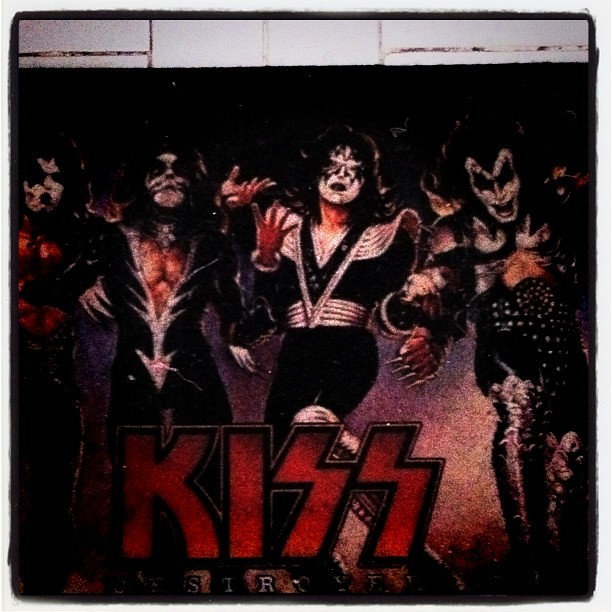This image features the iconic rock band KISS and appears to be an album cover, possibly for their "DESTROYER" album. The photograph, set against a dark background, prominently displays the band name "KISS" in bold red letters with black trim, the 'S's stylized like lightning bolts. Below the band's name, "DESTROYER" is inscribed in white lettering outlined in black. The four band members are centrally posed, all sporting their signature white face paint with distinct black designs. The first member on the left has a star over his right eye, the next member features cat-like makeup with whiskers and black around both eyes, the third member to the right has a mask-like silver and black outline around his eyes and nose, and the final member on the far right has demonic-style black makeup with an open mouth. Their outfits appear to be elaborate, possibly connected pantsuits, and include detailed elements like a long V-neck center and shoulder pads. The band members are gesturing excitedly or angrily with their hands, enhancing their rock persona. Light-colored cloth appears to reveal another texture behind it at the top of the image, though its exact nature is unclear.